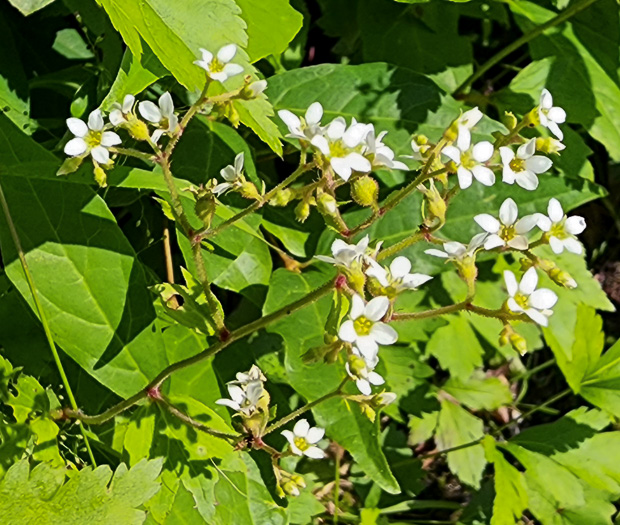This high-quality photograph captures a lush and densely green dogwood tree in full bloom outdoors. The tree's large, abundant leaves display intricate crevices and thick textures, with some variations in leaf types noted in the bottom left, bottom right, and along the top of the image. The vibrant greenery is bright and healthy, indicative of new growth. Emerging from the leafy backdrop are numerous stems that branch out, each adorned with several dogwood flowers characterized by their solid white petals, typically five in number, and striking yellow centers. The stems themselves exhibit a subtle, almost purplish hue where they separate. Among the fully bloomed flowers, there are also light green buds, some curled up, hinting at upcoming blooms or blooms that have recently dried up. This enchanting, detailed snapshot beautifully highlights the natural elegance and vitality of a dogwood tree in its seasonal splendor.